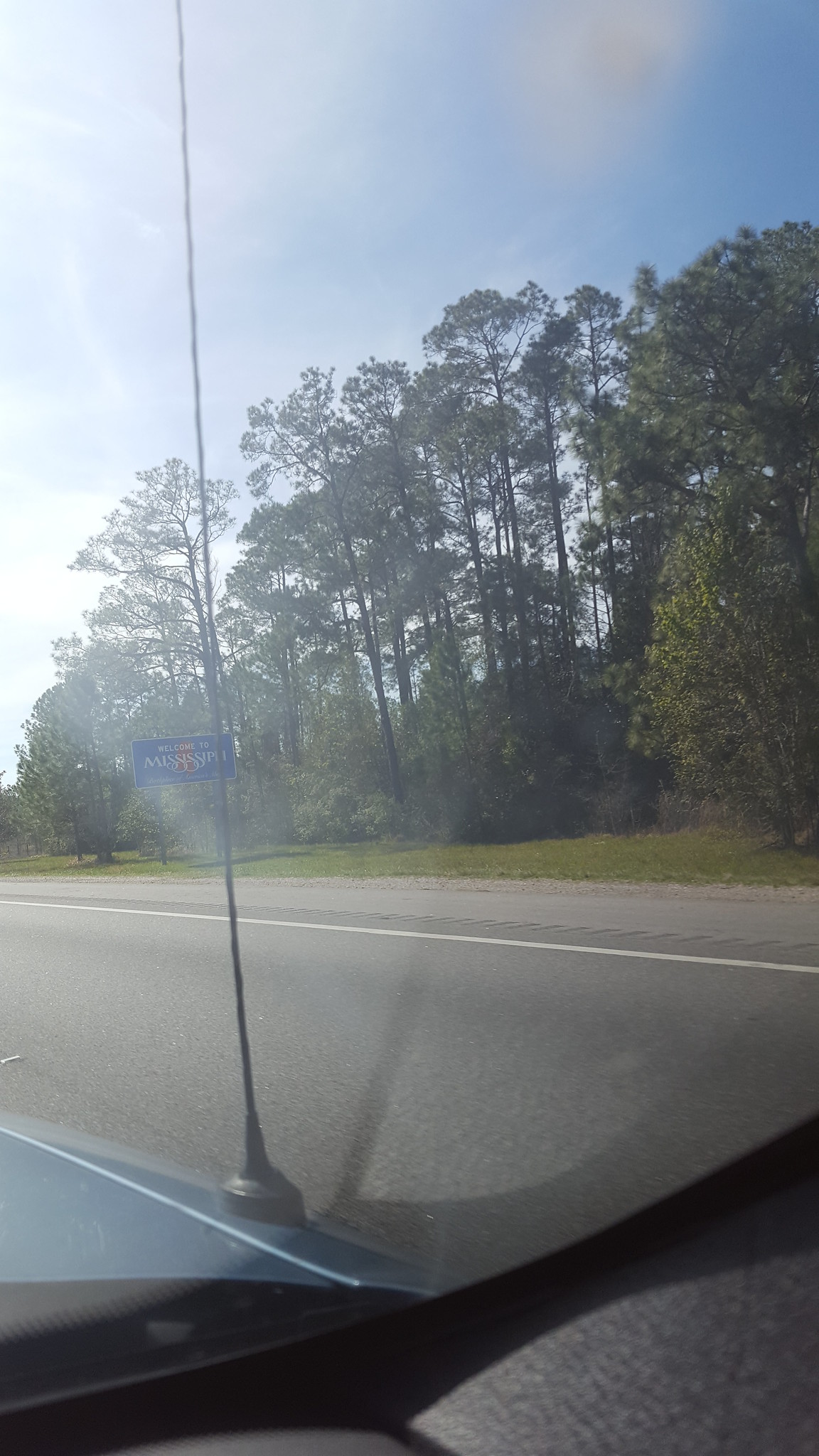A photograph taken from inside a car, capturing the view through a slightly hazy windshield. The perspective focuses on the car's hood, where an antenna cuts vertically through the frame. Beyond the car, a gray paved road extends into the distance, flanked by lush trees and patches of grass. Above, the sky is a clear blue peppered with wispy white clouds, indicating it is daytime. In the distance, a sign welcoming travelers to Mississippi is visible, marking the state's entrance.